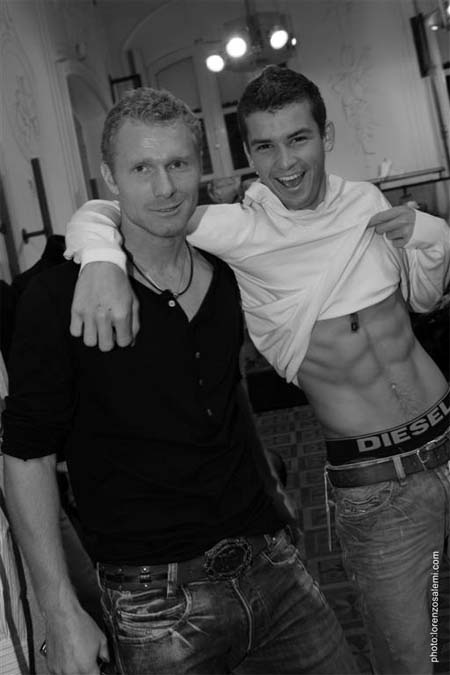In this black-and-white photograph, two young men, possibly in their 20s, pose together, radiating a sense of camaraderie. The man on the right, with dark brown, almost blackish hair, is lifting his white long-sleeved shirt to reveal a well-toned midsection, complete with visible abs. Beneath his lifted shirt, his black boxer briefs prominently display the brand name “Diesel” in light gray. Below his underwear, a brown belt cinches his lighter shade jeans. This man is smiling broadly, showing his teeth, and has his arm affectionately around his friend.

The man on the left, with short curly blonde hair, gazes directly into the camera with an assured expression. He is dressed in a dark, possibly black button-up shirt with the sleeves rolled up to his elbows, and a belt with a hexagonal buckle secures his jeans. A dark necklace or chain adds a hint of accessory to his outfit. Both men’s jeans are discernible despite the image's monochromatic scheme.

In the background, three lights, a window, and part of the walls can be seen, adding depth to the photograph. Additionally, the flooring and a small chandelier peek into the scene, contributing to the setting's ambiance. Adding to the personalized touch, the bottom right of the image bears the watermark “photolorenzosolemy.com.”